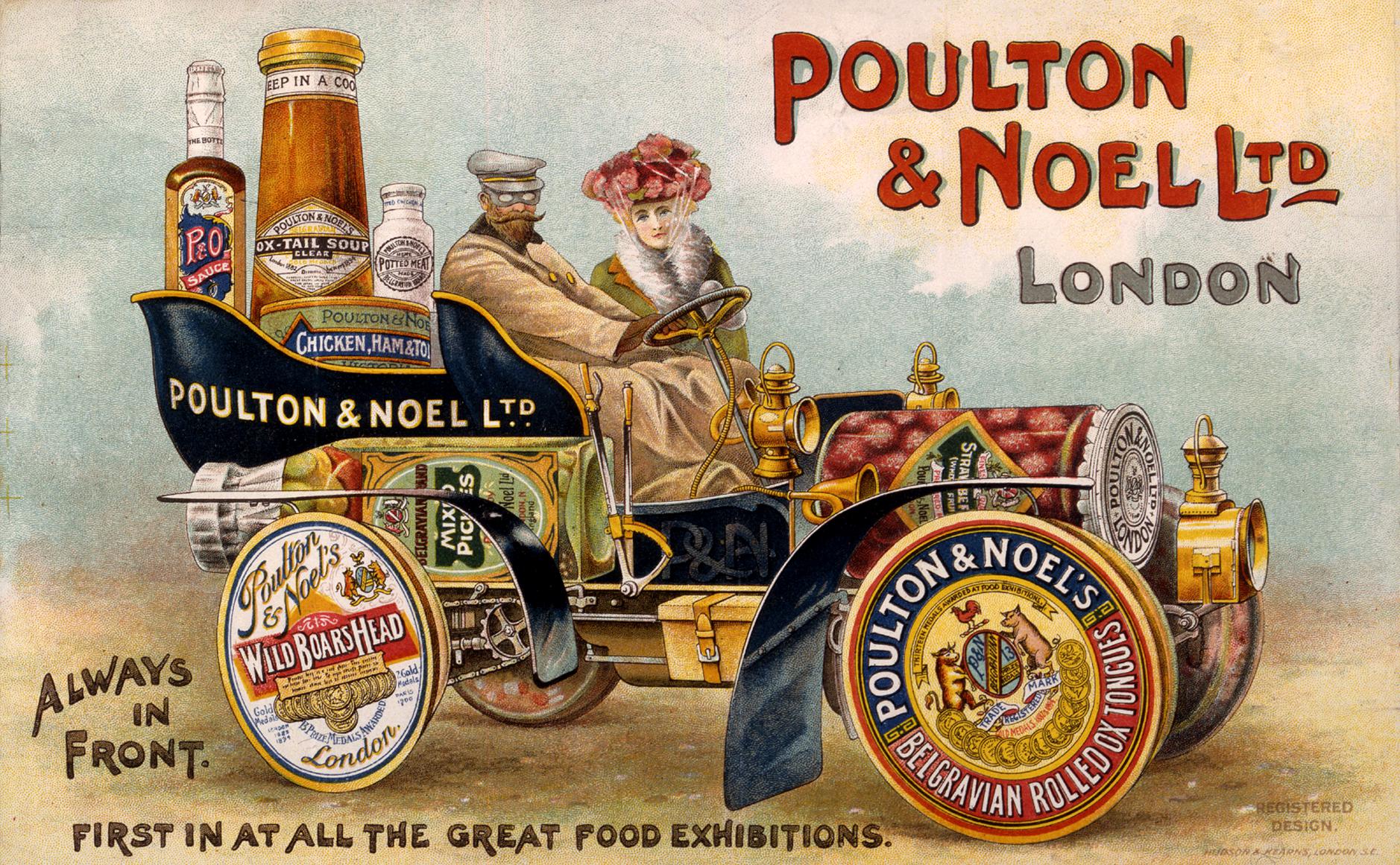This vintage advertisement for Poulton & Noel Limited, London, features a detailed hand-drawn illustration with text in distinct colors and styles. The brand name "Poulton & Noel" is prominently displayed in red vintage-style bubble letters in the top right corner, followed by "London" in gray text with a thin black outline and a light drop shadow. The tagline "Always in Front, First in at all the great food exhibitions" is positioned in the bottom left, written in black.

The central artwork portrays an old-fashioned open cabin vehicle ingeniously constructed from various Poulton & Noel food products. The wheels are round tins labeled "Poulton and Noel's Wild Boar's Head" for the back and "Poulton and Noel's Belgravian Rolled Ox Tongues" for the front. The back of the vehicle displays items like oxtail soup and possibly mixed pickles. A jar, perhaps containing a red circular product, is placed at the front tip of the vehicle, which is gold-colored.

Seated in the vehicle are a man and a woman, both dressed in period attire. The man, positioned on the left, wears a long beige trench coat, driving gloves, goggles, and a cap, and sports a distinctive curly mustache. The woman, on the right, dons a hat adorned with a bouquet of flowers and a fur coat tied under her chin with a bonnet. The depiction effectively showcases the diverse products of Poulton & Noel in a quirky and memorable setup.